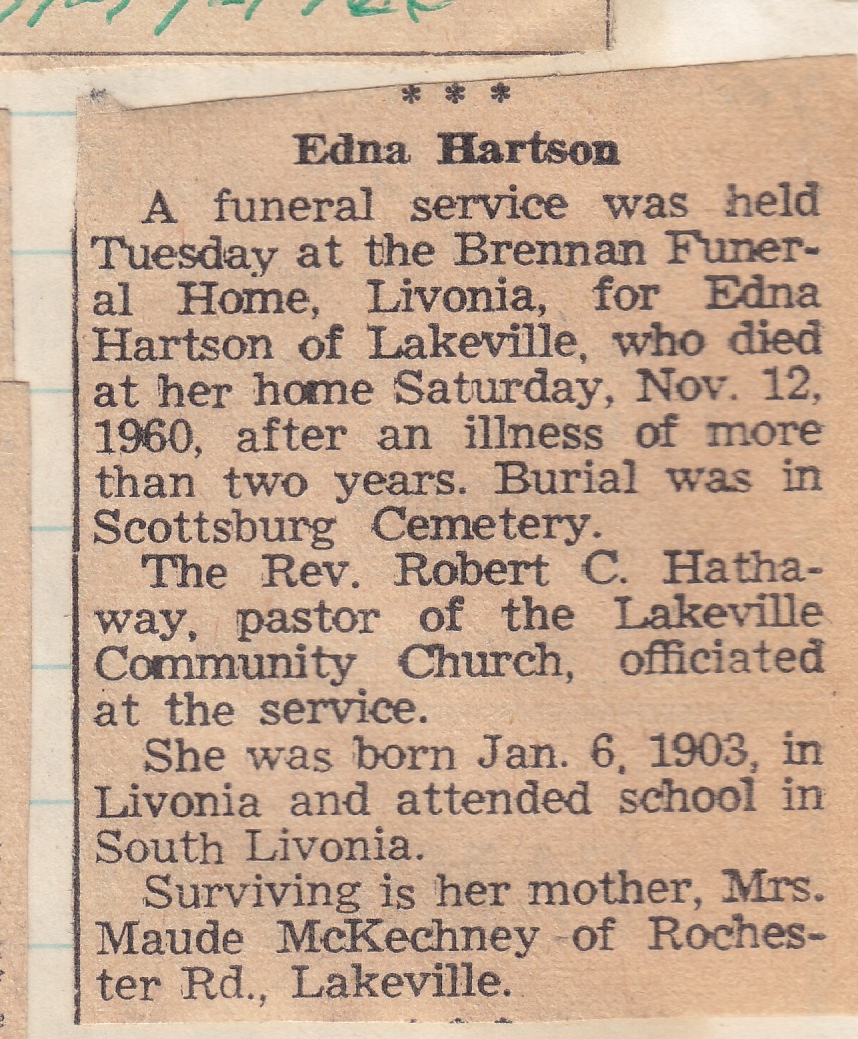This image appears to be a scan of an aged and discolored newspaper clipping, specifically an obituary for Edna Hartson. The clipping details that her funeral service was held on a Tuesday at the Brennan Funeral Home in Livonia. Edna Hartson, originally from Lakeville, passed away at her home on Saturday, November 12, 1960, after enduring an illness for more than two years. She was laid to rest in Scottsburg Cemetery, with the service officiated by the Reverend Robert C. Hathaway, pastor of the Lakeville Community Church. Born on January 6, 1903, in Livonia, Edna attended school in South Livonia. She is survived by her mother, Mrs. Maude MacKenzie, who resides on Rochester Road, Lakeville. This obituary, originating from the year 1960, shows considerable signs of aging, such as fading and discoloration, indicative of its historical nature.